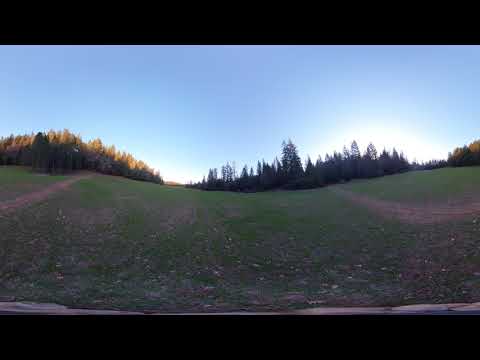This detailed image captures an expansive outdoor park during an autumn evening, either at sunrise or sunset. The grassy field occupies the lower half of the photo and features trodden paths with the dirt peeking through, suggesting well-worn trails. Slightly rolling hills add to the landscape’s gentle undulations. To the left, a cluster of deciduous trees displays their vibrant yellow fall foliage, while the right side of the image is flanked by verdant evergreen pine trees. The sky above is a clear, soft blue with few clouds, and the sun, setting or rising, casts a bright glow beyond the dense forest in the distance, giving the sky a dimly lit, dusky appearance. The upper half of the image is filled with the trees and the expansive sky. The absence of people and vehicles emphasizes the serene, tranquil nature of this picturesque scene.